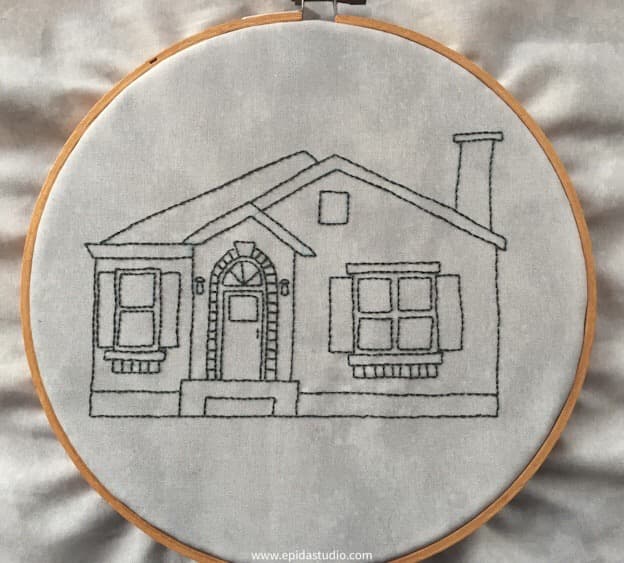This image captures an embroidery hoop featuring an unfinished piece of embroidery, set against a white material background. The hoop itself, a typical pine variety with a metal closure, encases fabric that has a marbled appearance with shades of gray and white. The embroidery, stitched in what appears to be dark, likely black, thread, outlines a traditional small house. Details of the house include two front-facing windows—a smaller single window on the left and a larger double window on the right. The house boasts a slanted roof with a chimney on the right side and an attic window near the roof. The front door is framed by brick detailing and features a single step stoop under a curved archway, adorned with two lanterns, one on each side of the door. Despite its charming aspects, the embroidery displays some signs of imbalance and asymmetry, indicating it is perhaps a work in progress or created by a less experienced hand. The overall scene lacks additional embellishments such as trees or a yard, placing full emphasis on the simplistic yet detailed portrayal of the house.